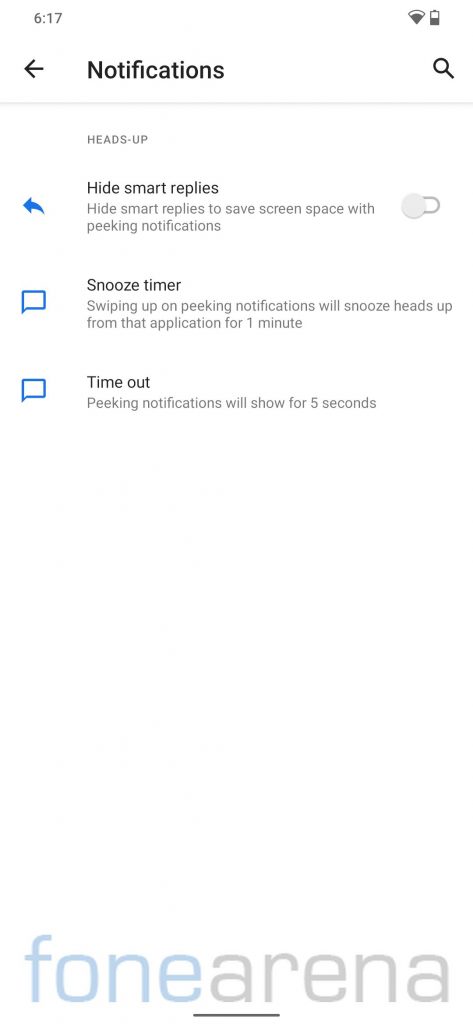The image is a cropped screenshot taken from a mobile device, showcasing the top half of the screen. It features a plain white background in the lower half and a watermark logo labeled "Phone Arena" at the very bottom, with "Phone" spelled as "F-O-N-E". The top section of the screenshot displays standard status icons indicating the time, Wi-Fi connection, and battery life. The main heading "Notifications" is centered at the top, flanked by a black back arrow on the left and a black magnifying glass search icon on the right. Below the heading, there are three notification management options listed: "Hide Smart Replies" with a toggle switch, "Snooze Timer," and "Time Out".